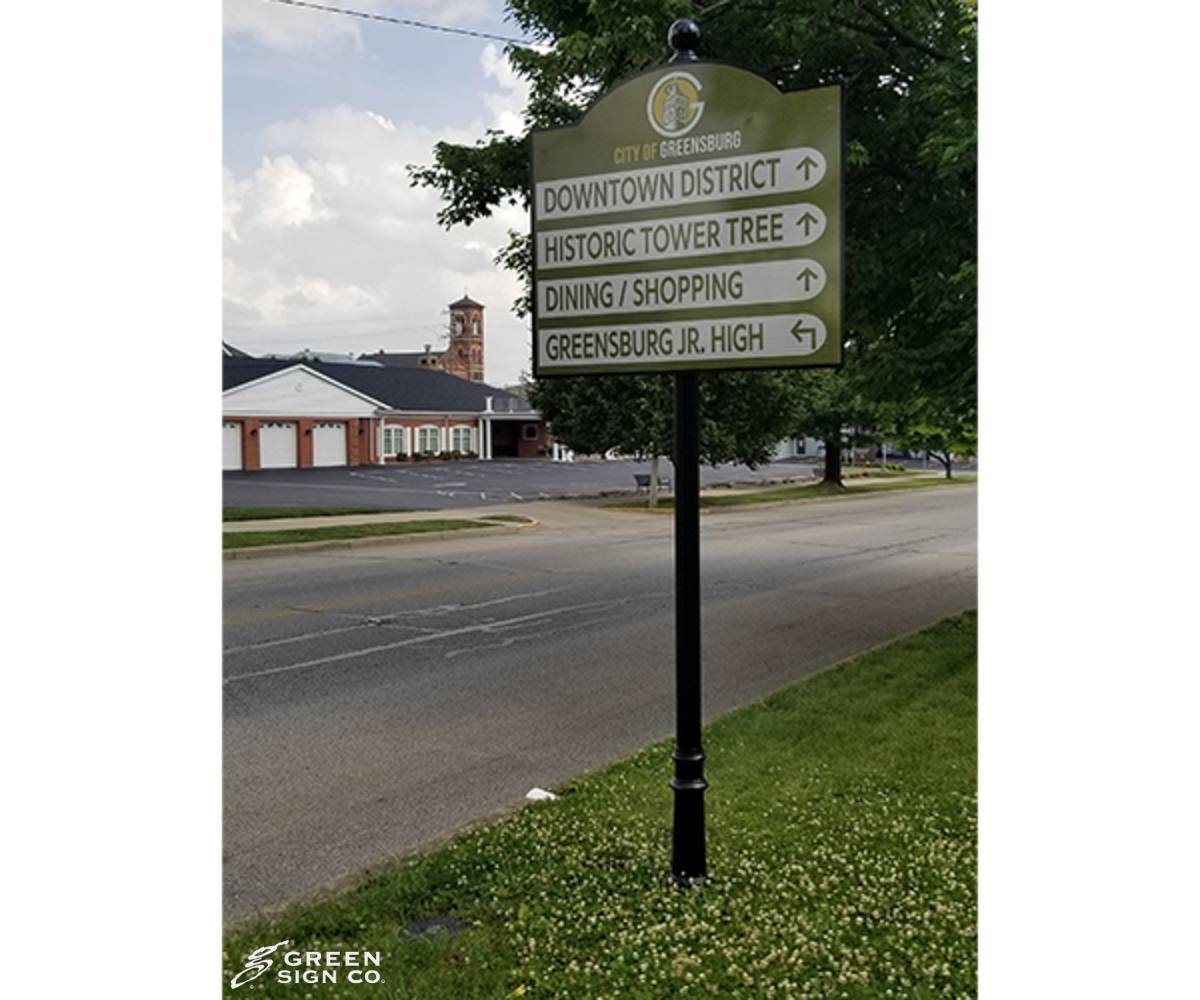The photograph captures a small town street scene in the City of Greensburg. Dominating the foreground is a prominent green sign mounted on a black pole. The sign features the text "City of Greensburg" in two shades of green and white, accompanied by a discernible logo with a "G" in white. Beneath the main heading, there are four directional indicators: "Downtown District," "Historic Tower Tree," and "Dining/Shopping," each with an upward-pointing arrow, and "Greensburg Junior High," which is directed to the left.

To the right side of the street, there is a stretch of grass and a noticeable tree. The left side of the street features a patch of grass, a sidewalk, and a brick building that stands one to two stories high with a black roof. In the background, towards the left, there's another building with a church-like steeple, possibly part of a funeral home parking lot with three visible garage doors. The scene is quintessentially small-town America, with an air of serenity and functional civic organization. The bottom left corner of the sign is marked by the Green Sign Company, indicating the craftsmanship behind the helpful landmark.